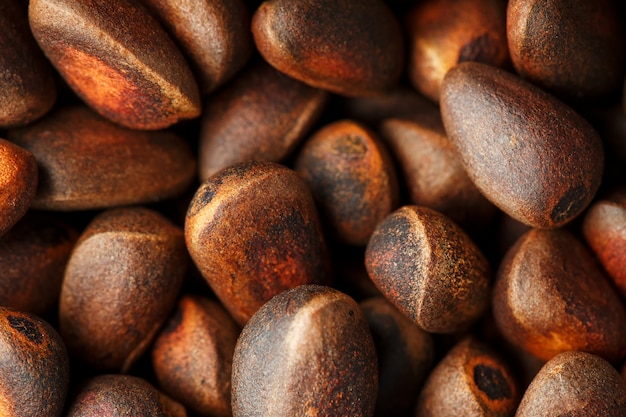Indoor color photograph showing an extreme close-up view of a pile of roasted walnuts completely filling the frame. The image captures approximately 25-35 walnuts, each exhibiting various shades of brown with a few having distinctive darker, almost black spots or seams. The composition offers no background or foreground details, focusing entirely on the walnuts, which are unbroken and stacked haphazardly. These nuts display a coarse, textured surface, enhanced by the roasting process that adds a hint of darker browning. The photograph, taken in natural lighting, features a palette of deep browns, with subtle light brown and yellow hues along some edges. No text or extraneous elements are present, emphasizing the simple yet rich detail of the walnuts.